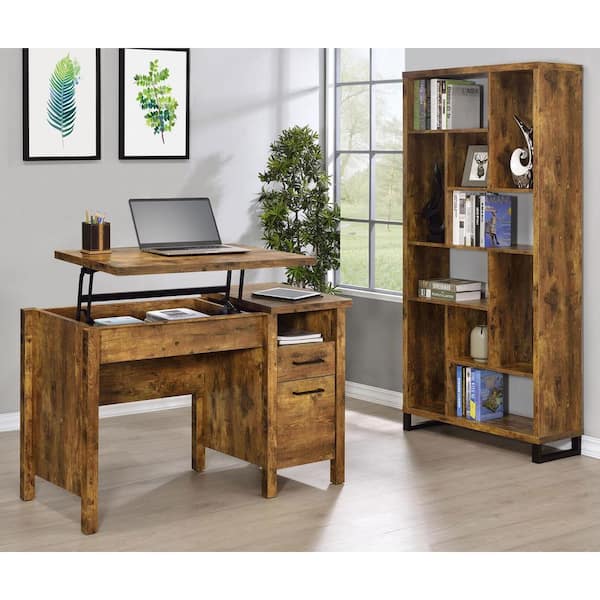This photograph captures a home office with a blend of natural details and functional furnishings. The central focus is a wooden desk, exhibiting a mix of brown tones, positioned in front of a light gray wall. On this desk, there's an open laptop with a gray screen, a tablet to the right of the laptop that appears to be a drawing tablet, and a box of tissues or potential stationery items. Two black-handled drawers and an open shelf holding two notebooks are on the right side of the desk. 

On the left part of the gray wall hang two framed illustrations: one depicting a green and blue leaf, possibly, and the other a branch with green leaves. Adjacent to the desk, to the right, is a window with eight panes, offering a view of trees and grass outside, hinting at a lovely backyard. Near this window in the corner sits a plant, approximately three and a half to four feet tall. 

The room also contains a tall wooden cabinet with multiple sections on the right side of the photograph. This cabinet houses books, decorative items, and a framed illustration of a goose. The floor appears to be a grayish hardwood, adding to the room's sophisticated yet cozy ambiance. Colors in the scene include shades of white, brown, green, blue, and yellow, contributing to a vibrant yet harmonious atmosphere.